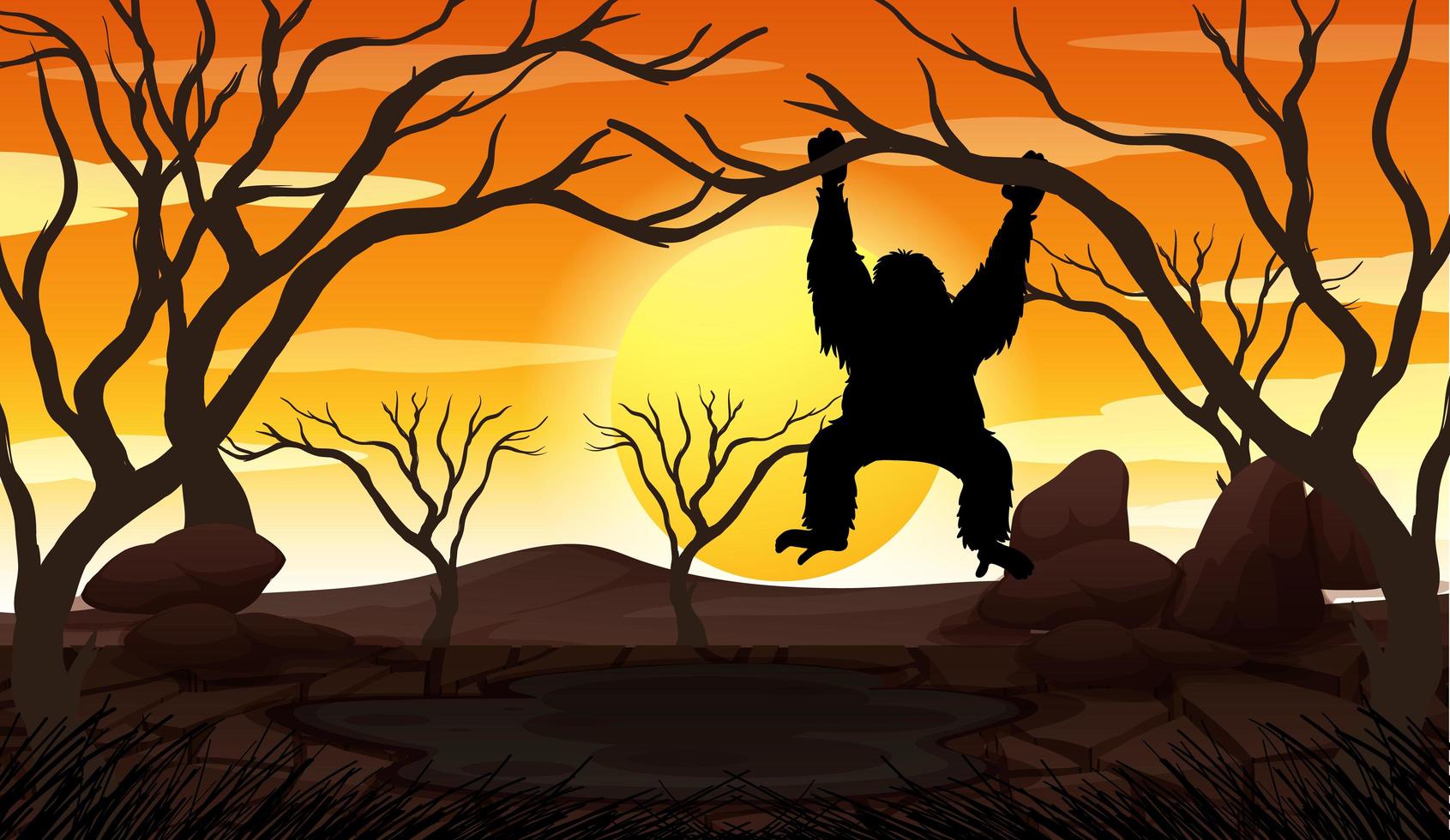The image is a detailed cartoon scene set during either a sunrise or sunset, characterized by a large, golden sun positioned on the horizon. The sun's glow transitions from a bright yellow at the base to a gradient of light to dark orange higher up in the sky, accompanied by a few white, wispy cartoon clouds. The foreground depicts a seemingly African or zoo-like setting, featuring three large, leafless trees with gnarled, veiny branches. A prominent silhouette of a monkey, possibly an orangutan, is seen hanging from one of the lower branches at the center of the image, its dark outline stark against the bright sun. The monkey's body and limbs are distinctly visible, emphasizing its furry texture. Below the monkey and to its right, the ground is shaded and dotted with several large rocks. The scene has a horizontal composition, with additional trees and a gentle hill further in the background, creating a picturesque and serene landscape. The overall aesthetic is cartoonish, vividly capturing the essence of the setting through silhouettes and bold colors.